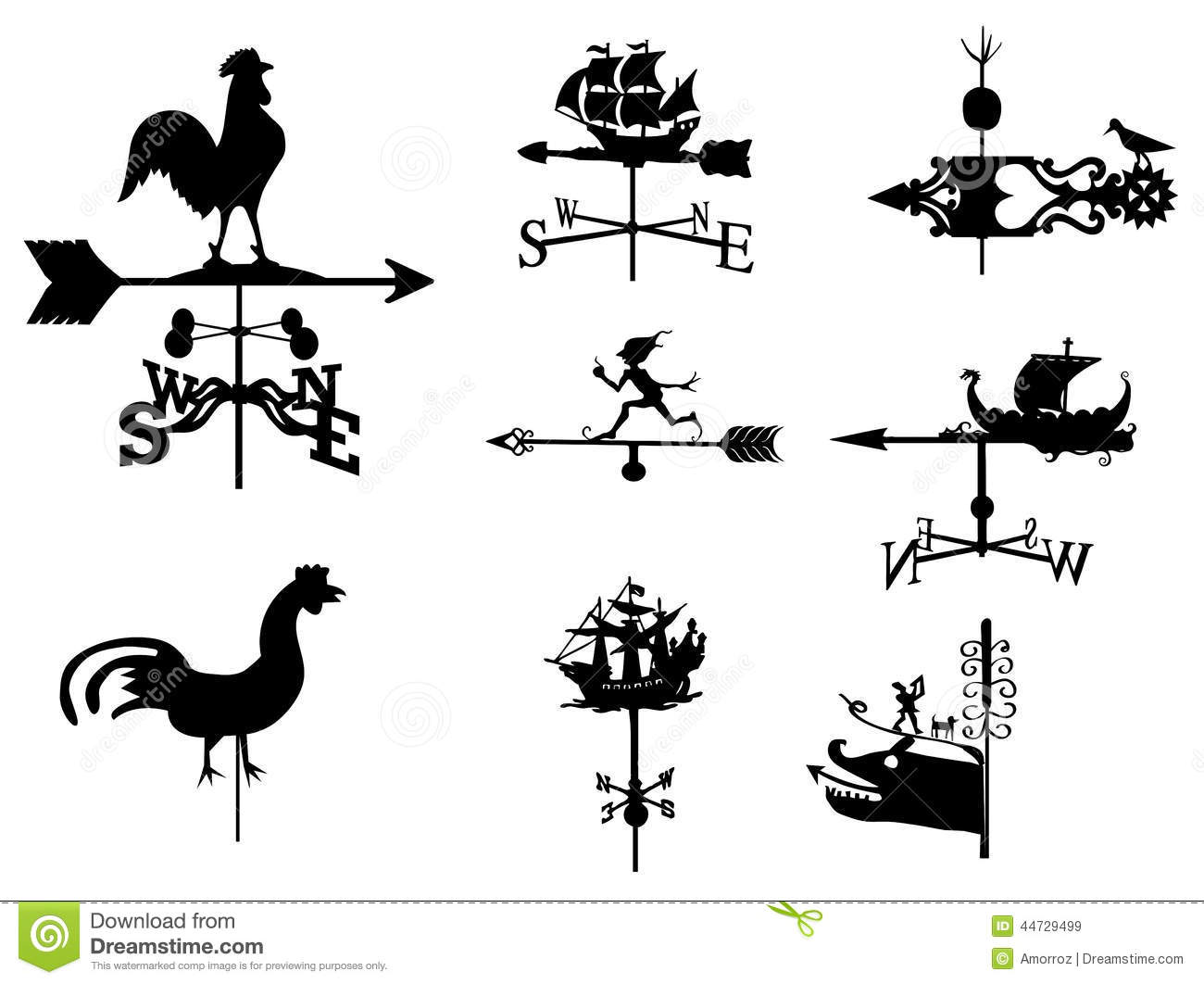The image showcases eight detailed black weather vanes set against a white background, presented in a stylized, drawn format. The top left corner features a classic rooster weather vane with directional indicators (N, E, S, W). Below it is another rooster vane, though this one lacks directional letters. The top middle vane depicts a traditional ship with four sails, flanked by single sails on each side. Adjacent to it is a more intricate design featuring a gear, a bird outline, and a circle. In the middle row, the left vane includes the directional letters without a topper. The central vane showcases a running figure, while the right vane illustrates a ship with one large sail. The bottom row begins with another rooster vane on the left, followed by a simple ship vane in the middle, and concludes with a whimsical whale vane on the right. Throughout the image, faint spiral watermarks and gray lines are evident, along with an embossed green arrow indicating it's sourced from dreamstime.com.